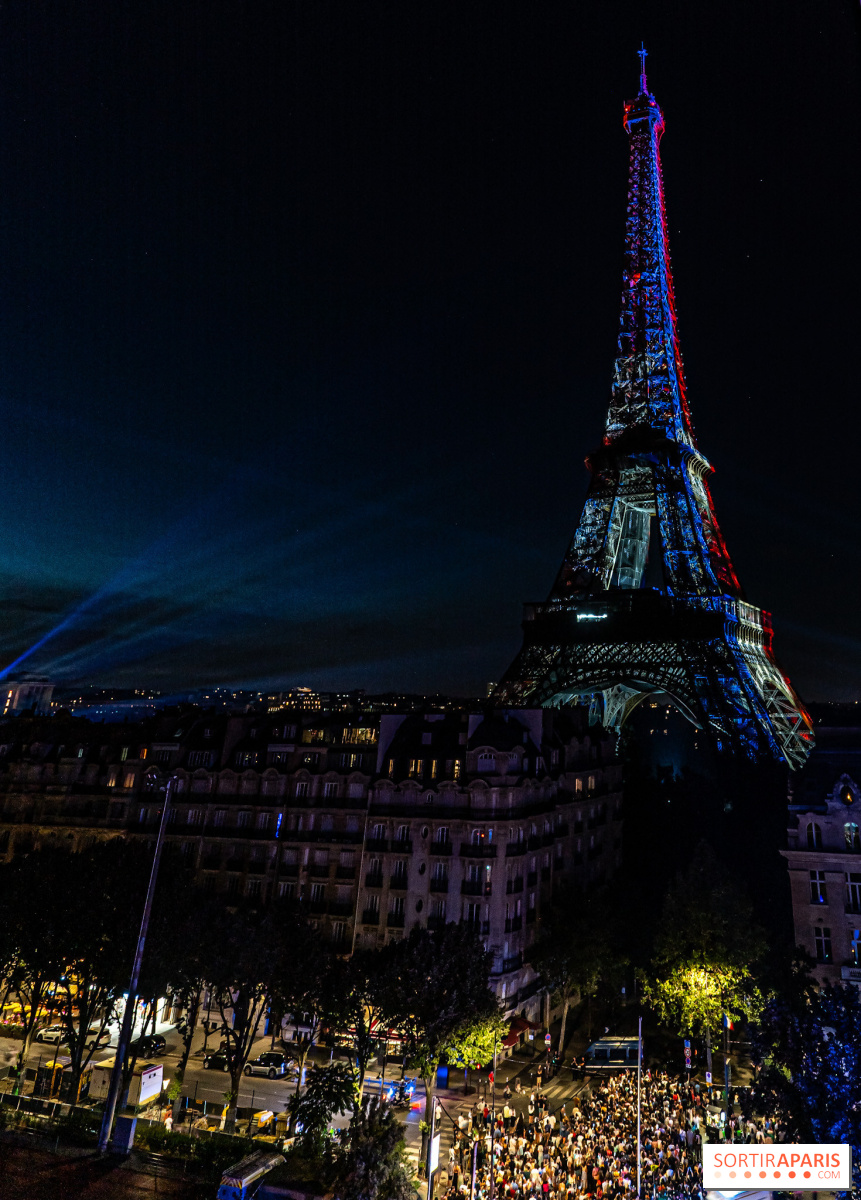A captivating photograph of Paris at night, centered on the vibrant Eiffel Tower. The iconic structure, bathed in stunning purple and blue lights with a brighter blue midsection, dominates the right side of the image, set against an ink-blue sky where a few faint stars are visible. Taken from a distance, the perspective includes several apartment buildings at the tower's base, hinting at the residential area. In the lower right corner, the coral pink logo "Sortirapierie" is visible, accompanied by a crowd of people gathered on a dimly lit street, enhancing the urban night scene. To their left, a relatively empty street illuminated by streetlights and car headlights adds depth to the composition.